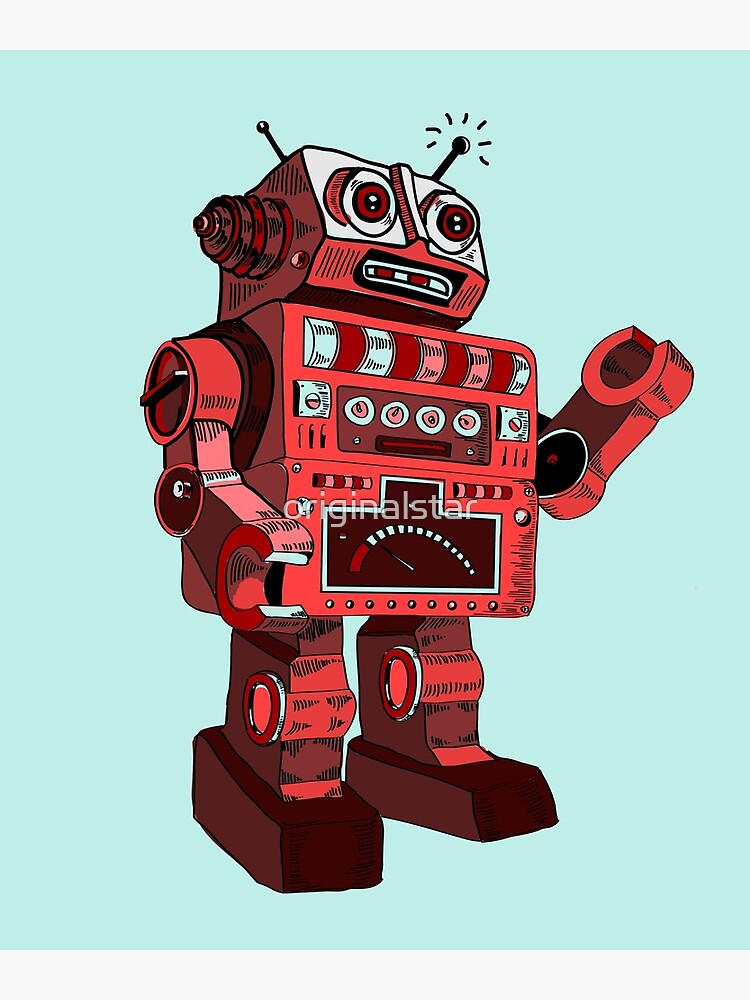The image is a detailed drawing of a vintage toy robot set against a light teal, almost turquoise, background. The robot is predominantly red and has a boxy, rectangular design, where the left and right sides of the rectangular image are twice as long as the top and bottom sides. There is a thin gray border at the top and bottom of the image. The robot, facing rightward, is characterized by its square head, which features two small antennae, two eyes, a small nose, and a mouth shaped like a cassette tape opening.

The robot's torso is also box-shaped and adorned with multiple lights, various gauges, and a circular dial. Its arms terminate in large, C-shaped claws that appear unable to close fully. The legs are mechanical with structures resembling cylinders at the knees. The feet are dark red and rectangular, seemingly solid and robust. The overall design presents a vintage aesthetic through its detailed, almost mechanical features and vibrant coloring.